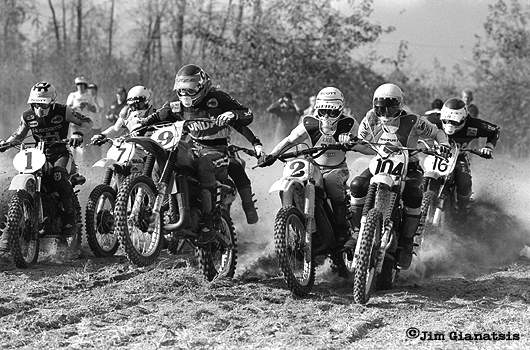This is a detailed black-and-white photograph capturing an intense motorbike race on a dusty field. The image shows eleven, possibly twelve participants, with several identifiable motorcycles bearing numbers such as 1, 7, 9, 2, 104, and 16. The motorcyclists are all wearing helmets and are equipped with both darker and lighter colored jackets. In a dynamic moment, the rider on bike number 9 is seen doing a wheelie, with the front tire lifted off the ground. The race seems to be taking place in a field that has a grassiness mixed with hay texture, given the grayscale nature of the photo. Spectators and photographers, some of whom are helmetless, are visible in the background, against a backdrop of trees and sky. Smoke and dust are being kicked up by the moving motorcycles, highlighting the speed and energy of the scene. The photograph is credited to C. Jim Giannatissis, whose signature appears in the lower right corner.